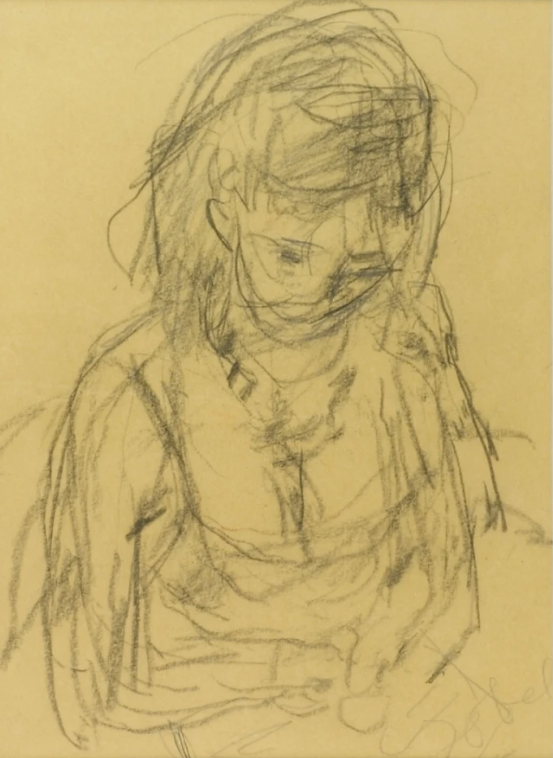The image portrays a vertical rectangular sketch of a young girl rendered on dark yellowish-brown paper. The rough, loose lines of the brown or charcoal pencil give the sketch a dynamic, almost chaotic feel, reminiscent of the Pig-Pen character's aura from Charlie Brown. The girl, appearing about ten years old, looks downward, with shoulder-length, messy hair and noticeable bangs. Her facial features, though indistinct, show subtle curves for eyebrows and shaded areas for her eyes, suggesting movement and emotion. She seems to be wearing a dress with thin straps originating near her armpits, and her hands are folded in her lap, visible down to her waist. Various random lines and textures surround her figure, adding to the sketch’s overall sense of motion. In the bottom right corner, there's a cursive signature, possibly by the artist, but it is unreadable.